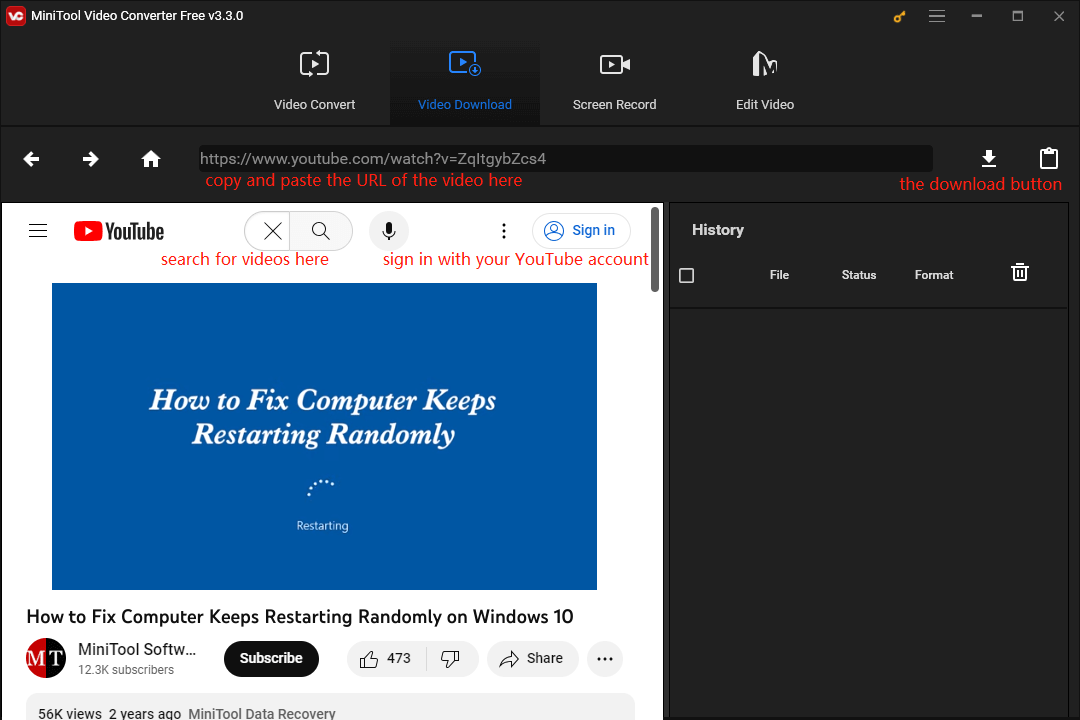This image appears to show a computer screen, possibly a screenshot taken by someone experiencing issues with their system and seeking solutions online. The main focus of the image is a YouTube video tutorial that appears on the left-hand side. The top right corner of the screen shows a black background with a window titled "MiniTool Video Converter Free." The user has clicked on the "Video Download" option within this software.

Dominating the left side is a pop-up YouTube video interface, neatly framed with a white border. Within this interface, there is a blue rectangle in the center that contains white text reading "How to fix computer keeps restarting randomly." Below this, a loading indicator is visible with the word "restarting" next to a spinning loading icon, suggesting the user's computer is in the process of rebooting.

Further down, the text reiterates the video's title, "How to fix computer keeps restarting randomly on Windows 10," followed by an attribution to MiniTool software, abbreviated as "MT." Below the video title, a blue 'Subscribe' button is present, indicating that users can subscribe to the channel for more content. It is unclear whether the subscribe button has been clicked in this image.

Overall, the screenshot effectively captures a moment where the user is actively troubleshooting their computer issue by watching an instructional YouTube video while interacting with a video conversion tool.